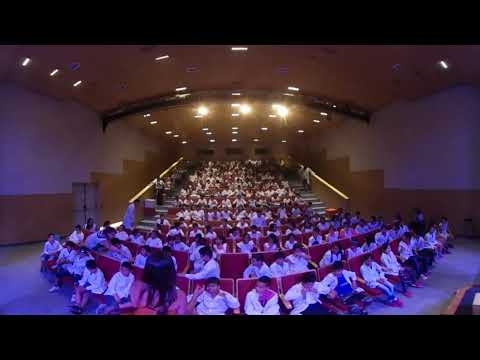The image depicts an auditorium or lecture hall from the perspective of the stage. The venue features tiered seating that arches in a U-shaped formation, gradually rising toward the back. The walls of the hall are a combination of white and brown, with the brown section primarily at the bottom. The arched ceiling, also brown, is illuminated by multiple spotlights, including three prominent ones near the front.

The students, clad uniformly in white jackets, appear to fill every seat. Notably, a girl in a pink outfit with long, dark hair sits at the front. Another young woman, partially visible at the bottom of the image facing the crowd, seems to be explaining something with her arm slightly raised. Spotlights and gold or white ceiling lights provide illumination, contributing to the ambiance of the space. The entire scene is framed by horizontal black bars at the top and bottom of the image, emphasizing the panoramic view of the auditorium.